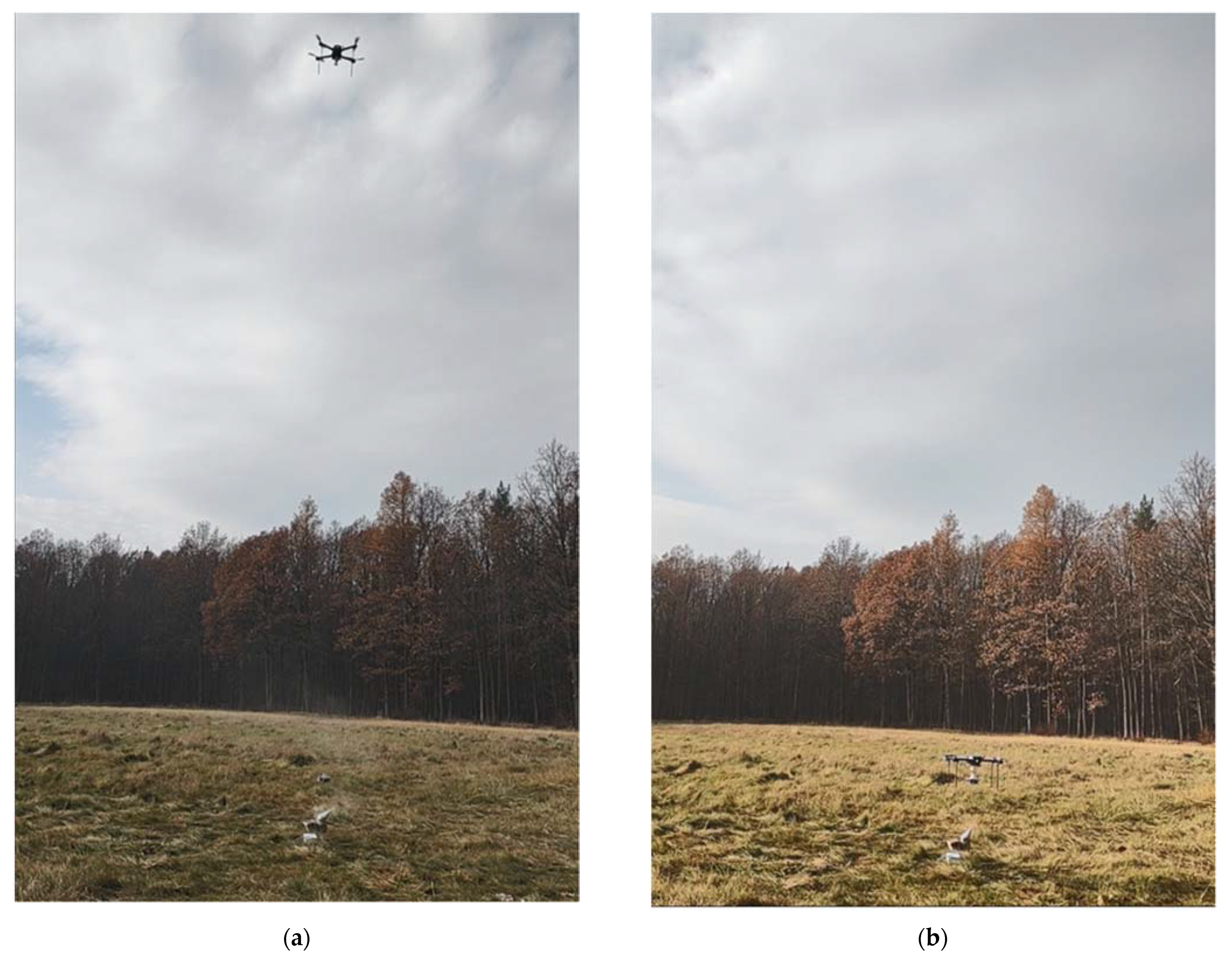The image features two vertically rectangular photos, labeled "A" and "B" at the bottom, placed side by side against a white background with a thin white strip separating them. Both images depict a grassy field set against a dense line of trees, with signs of autumn foliage. The sky is overcast with a mass of gray-tinted, fluffy white clouds. 

In image A, situated on the left, a black drone with small wings is captured mid-flight against the cloudy sky. A faint plume of smoke or dust marks its takeoff spot on the ground below. Image B, on the right, shows the same drone hovering just above the grass near its takeoff location. The colors in image A appear slightly darker compared to the brighter hues in image B, making the grass and trees seem lighter in the latter. The overall composition emphasizes the drone's journey from airborne in image A to nearly landed in image B, with consistent natural elements framing the scene.